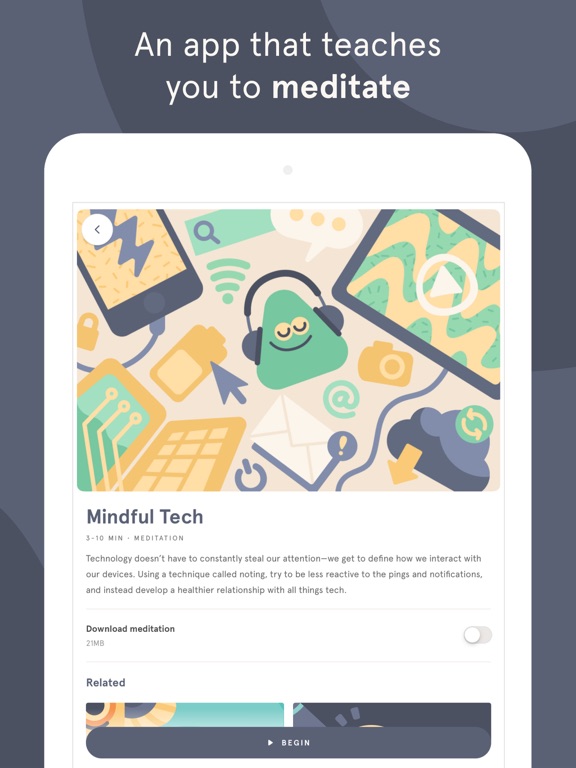Promotional Advertisement for Meditation App:

Set against a dark purple, almost gray background, this promotional image highlights a meditation app designed to help users find tranquility. At the top of the image, white text announces, "An app that teaches you to meditate." Below this text, a tablet-shaped device with a white outline and a pinhole camera at the top is prominently displayed.

On the simulated tablet screen, the app interface features a large, anthropomorphized triangle character with rounded edges. The cheerful triangle, adorned with headphones, smiles serenely, symbolizing the peace and joy brought by the app. Surrounding this main character are other whimsical cartoon images of cell phones, tablets, laptops, and notification symbols, emphasizing the app's integration with various devices.

Beneath the tablet mock-up, additional text reads, "Mindful Tech: 3 to 10-minute meditations. Technology doesn't have to constantly steal our attention. We get to define how we interact with our devices." This closing statement reinforces the app’s mission to help users reclaim their focus and interact with technology in a mindful manner.